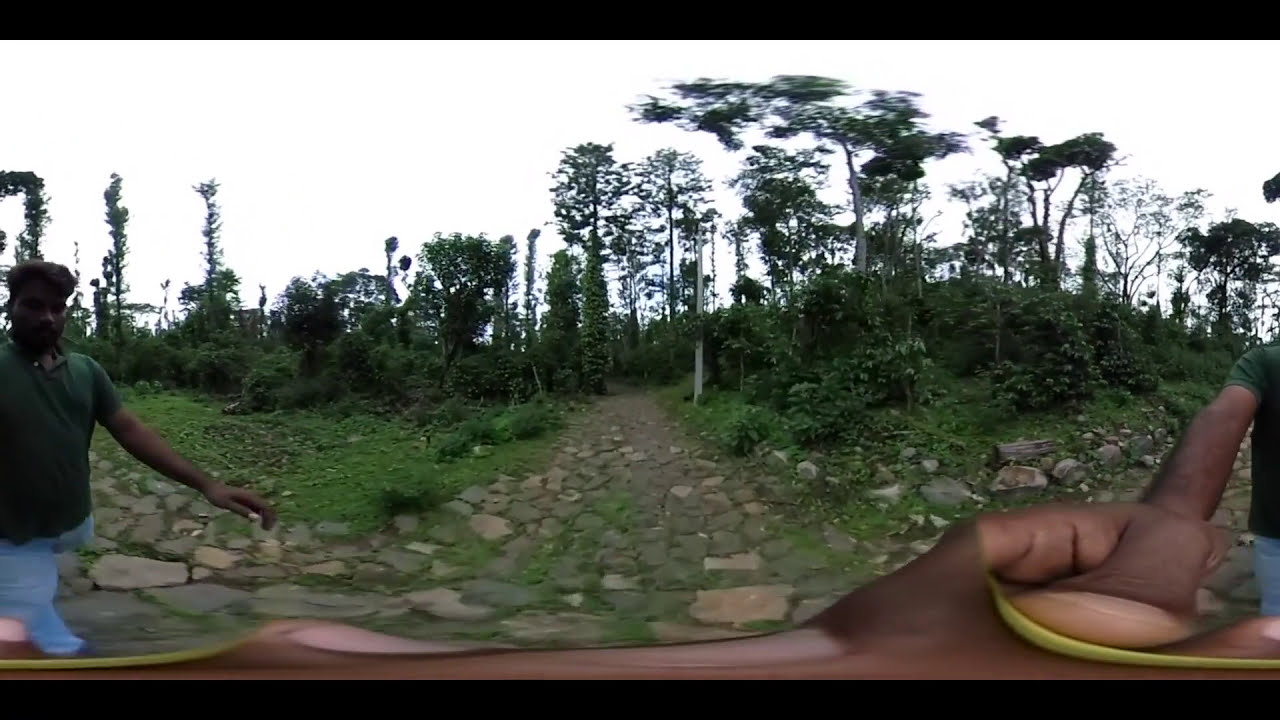The image depicts a panoramic, possibly fisheye-lens view of an outdoor scene, potentially a park, characterized by a central stone path that appears to extend both horizontally and into a dense, green forest. The path, composed of light and dark brown cobblestones intermixed with dirt, is bordered by grass, small shrubs, and bushes that gradually transition into taller trees and ivy as they recede into the background. The sky is overcast, appearing bright but white and gray. On the left side of the path, a man with dark skin and dark hair, dressed in a dark green short-sleeved T-shirt and light blue jeans, is walking. Interestingly, a similar figure, possibly the same man, appears on the right side of the image, suggesting a distortion typical of a panoramic photo. Additionally, a distorted hand, presumably the man's holding a camera, stretches along the bottom of the image.